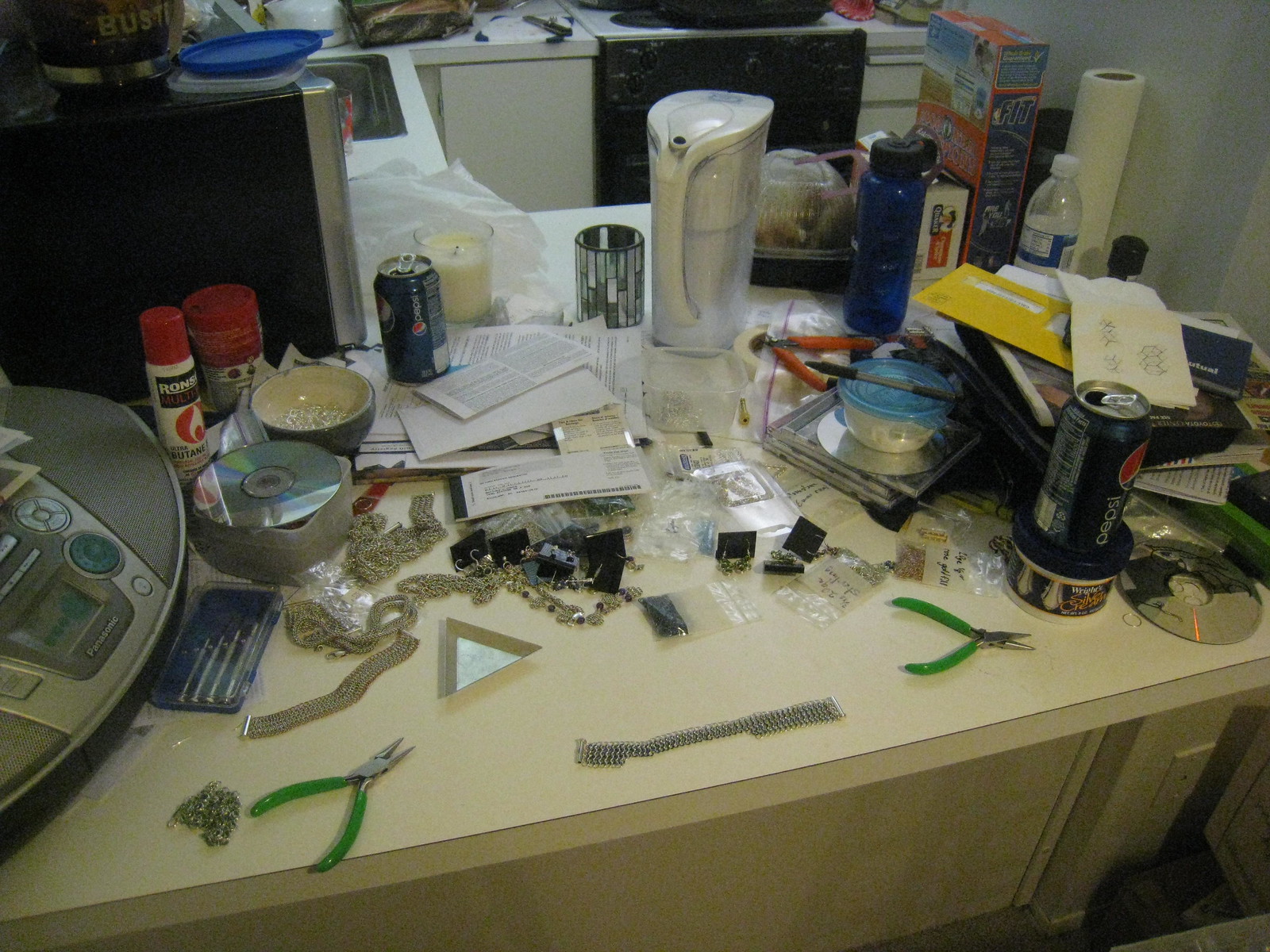The image depicts a cluttered kitchen table and countertop. The countertop has a tan, off-white linoleum surface. To the left side of the countertop, there is a stereo boombox with a CD placed on a small shelf next to it and a can of butane fuel nearby. An open can of Pepsi sits atop a stack of open mail. Below that, a collection of unclasped chains, necklaces, and bracelets are scattered about, some in small plastic baggies. Two pairs of needle-nose pliers with green handles, several pens, a Brita water filter, a plastic water bottle, and another open can of Pepsi on top of a container are also visible. To the right, there is a container on a stack of CDs, next to a pen.

In the background, the kitchen area features a stove with another counter and a sink to the left. A microwave on the left side of the image partially obscures this view. Scattered around the scene are a couple of candles, a roll of paper towels, a container of laundry detergent, unopened mail, a napkin with doodles, and various small pieces of packaging. The overall impression is one of disarray, with numerous items haphazardly spread across the surfaces.